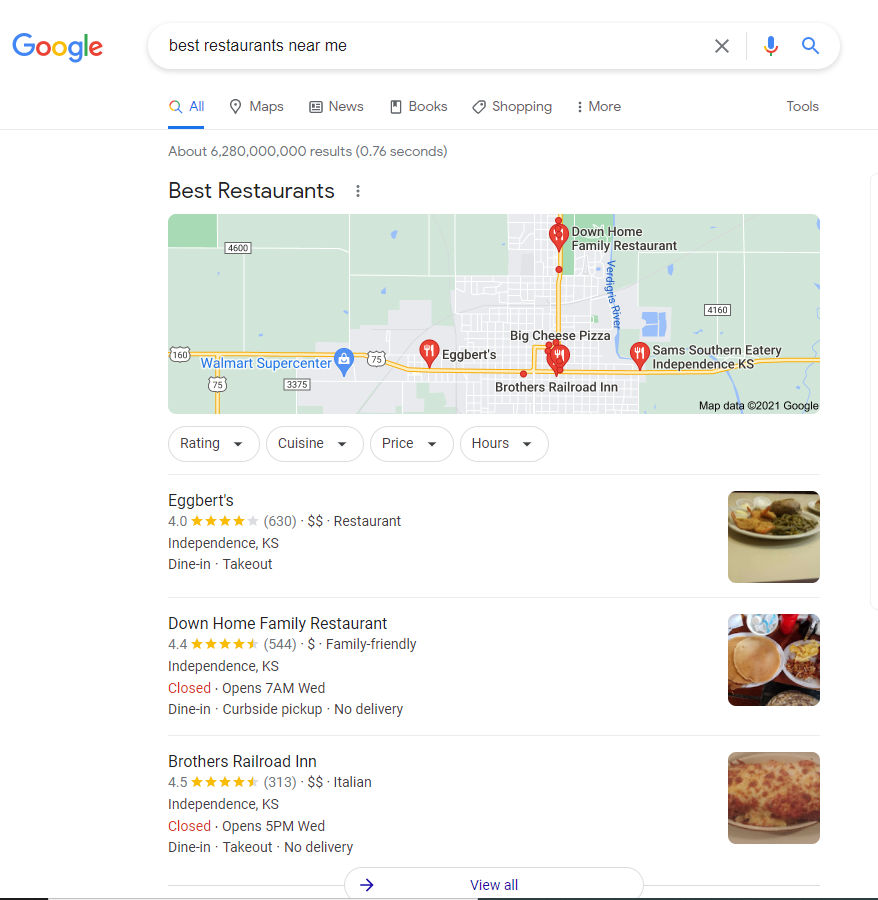The image displays a Google search results page. At the top left, there is the iconic Google logo, featuring a blue "G," a red "O," a yellow "O," a blue lowercase "g," a green "l," and a red "e." To the right of the logo is the search query field, an elongated oval shape currently containing the text "best restaurants near me" in black font. Adjacent to the search field on the right, there is a gray "X" for clearing the search text, followed by a short, light blue vertical line divider. Further right, there is a colorful microphone icon in Google’s colors, and next to it, a blue magnifying glass icon angled towards the left with its handle pointing downward to the right.

Below the search bar, the navigation options "All," "Maps," "News," "Books," "Shopping," followed by a menu denoted by three dots and the "More" option appear in light gray text. The "All" option is highlighted in blue with a bold blue underline indicating it is currently selected. To the far right of these options, the "Tools" menu is also visible.

Just below this navigation menu, there is a line of small gray text that states "About 6,280,000,000 results (0.76 seconds)," indicating the number and speed of the search results. Below this, in larger black font, the search query "best restaurants" is displayed. To the right of this text, there are three vertically aligned black dots.

Below the search information, a large rectangular map with various map pins representing different locations is shown. Beneath the map, there are four oval-shaped filter options with light gray borders, labeled "Rating," "Cuisine," "Price," and "Hours," each accompanied by a downward-facing arrowhead indicative of a dropdown menu for further filtering options.